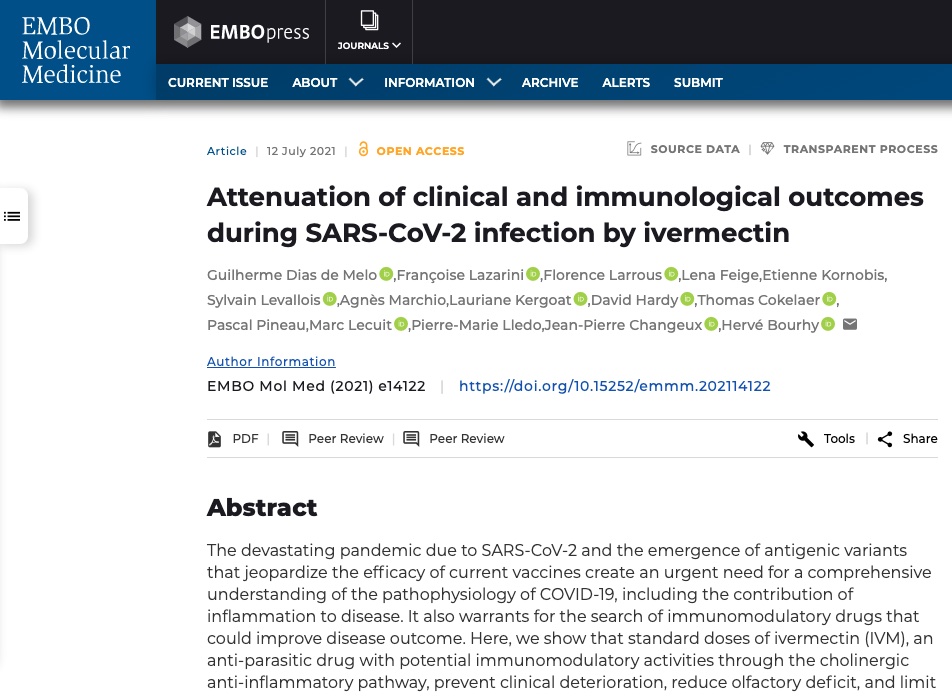Screenshot of the EMBO Molecular Medicine webpage on a white background. The header displays the names “EMBO Molecular Medicine” and “EMBO Press,” along with navigation links such as “Journals,” “Current Issue,” “About,” “Information,” “Archive,” “Alert,” and “Submit." Below the header, there are three rectangles containing three smaller squares each. The main section features an article titled "Attention of Clinical and Immunological Outcomes During SARS-CoV-2 Infection by Ivermectin," dated July 12, 2021, marked as Open Access with available Source Data and a Transparent Process.

Authors' information is listed, highlighted in blue, and linked to additional details. Citation details read "EMBO Mole Med 2021, EL4122." The page includes functionality links for "PDF," "Peer Review," "Peer Review 2s," and "Share." The article abstract is present, and multiple blue hyperlinks provide further access to extended content and resources.